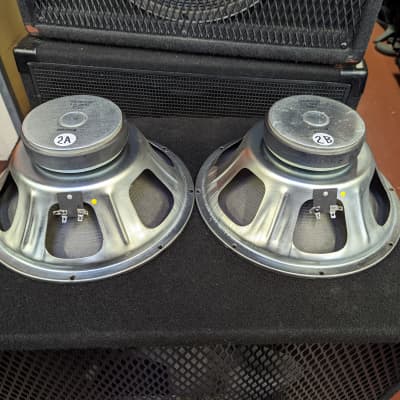In front of me is a detailed close-up image featuring two silver mechanical parts of speakers labeled "2A" and "2B." These components, likely intended for car installation or similar purposes, are placed upside down atop a larger black self-contained speaker housed in a box. This larger unit appears to be a woofer, potentially part of an amplifier setup. Behind this arrangement, additional equipment is visible, including another speaker and a case suggesting a storage or display function, possibly for sales purposes. The scene is set against a brownish-orange floor, with the faint presence of shoe-clad toes in the upper right corner, adding a human element to the otherwise technical display.